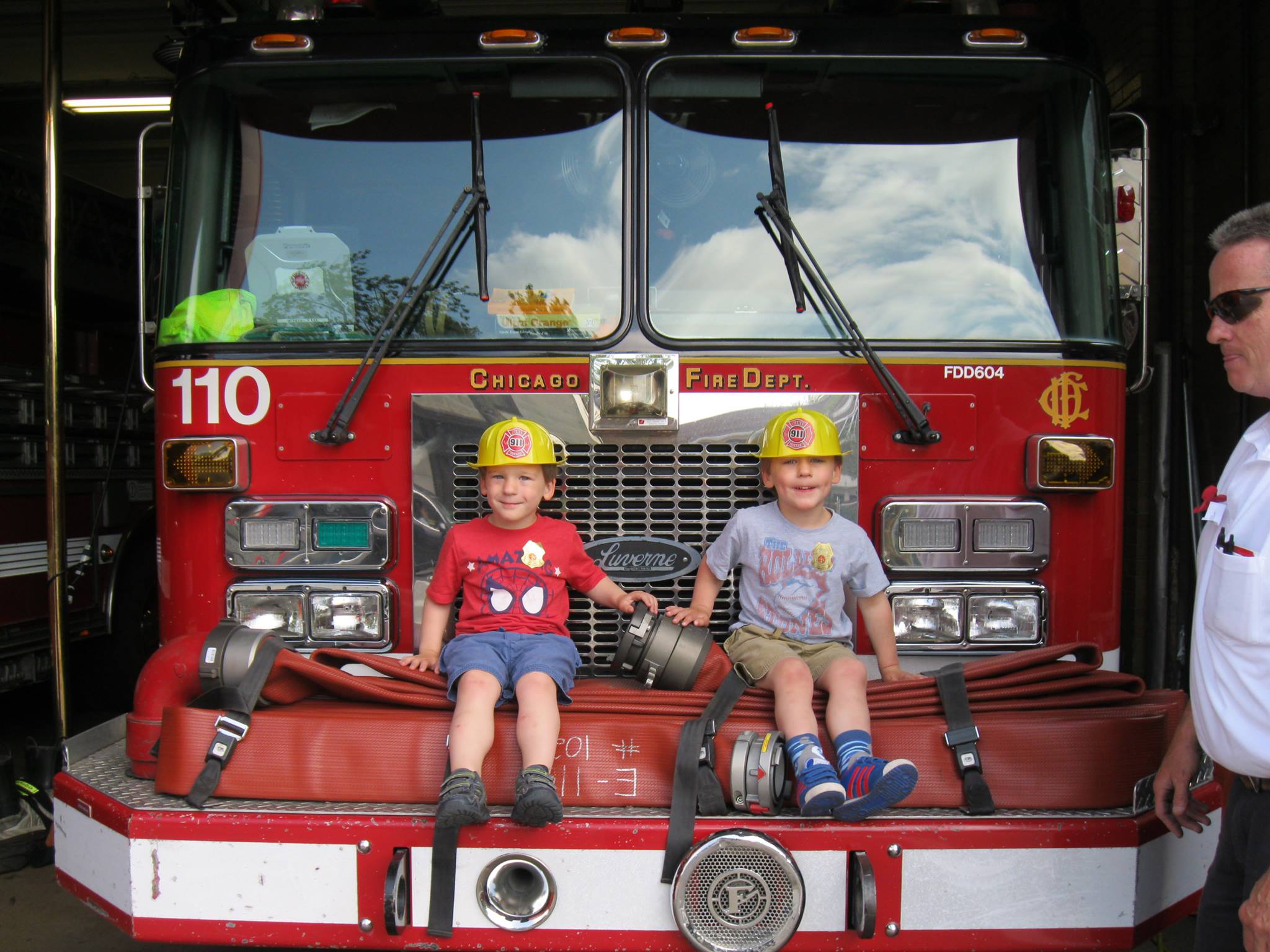In this vibrant photograph capturing a "Meet the Fire Department" day with the Chicago Fire Department, we see two small boys sitting happily on a large folded-up fire hose at the front of a red firetruck labeled with "Truck 110" on the left side in white. Both boys are wearing yellow toy firemen helmets. The boy on the left dons a red Spider-Man shirt, blue shorts, and black shoes, while the boy on the right sports a gray shirt, khaki shorts, and blue adidas shoes. They appear to be twins, sharing similar looks and joyful expressions. Situated near the front of the firetruck, a fireman stands closely observing them, wearing sunglasses and a dress shirt with pens neatly tucked in his chest pocket. The firetruck is equipped with two windshield wipers on each of the large windows, and a laptop is visible inside the cabin. The bright, sunny day adds to the cheerful atmosphere as the boys enjoy their special moment, with this candid shot likely taken by their proud parents as a keepsake.